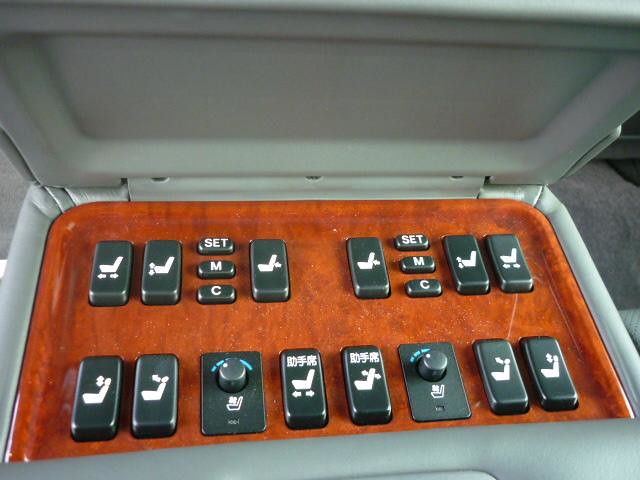This image is a close-up photograph of a control panel, possibly from a mini-passenger van or another type of vehicle with reclinable seats. The control panel is housed inside a gray plastic or upholstered case with a propped-open lid, revealing the controls situated on a shiny darker wood background. Surrounding the controls is gray leather trim. The panel features various black buttons and knobs, many of which have icons depicting seats with directional arrows, indicating that the buttons adjust the seat positions, including moving the seats forward, backward, upward, and downward. Notably, there are additional buttons labeled "Set," "M," and "C." Some of the buttons and dials bear Chinese or other Asian-language characters. The arrangement also includes a dial, likely for adjusting the heating or cooling functions in the seats. The precise functionality of each control is not entirely clear from the image alone, but the panel seems equipped to manage multiple seat and climate settings.